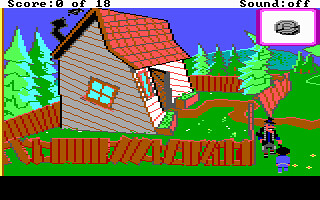Captured in a pixelated, retro video game style, this image portrays a dilapidated house viewed from the side. The house, clad in beige siding and topped with a red, sagging roof, appears to lean slightly askew, adding to its rundown appearance. A single, centered four-pane window pierces the side wall, hinting at neglected interiors. The house is nestled within a fenced grassy yard, enclosed by a deteriorating wooden board fence. Majestic evergreen trees rise in the background against a clear blue sky, contrasting the house's shabby state. In the bottom left corner, outside the fence, two characters can be seen, likely player avatars. An informational overlay at the top of the image reads "Score: 0 of 18" and "Sound: OFF" in black text, framing the scene within the context of an ongoing game.